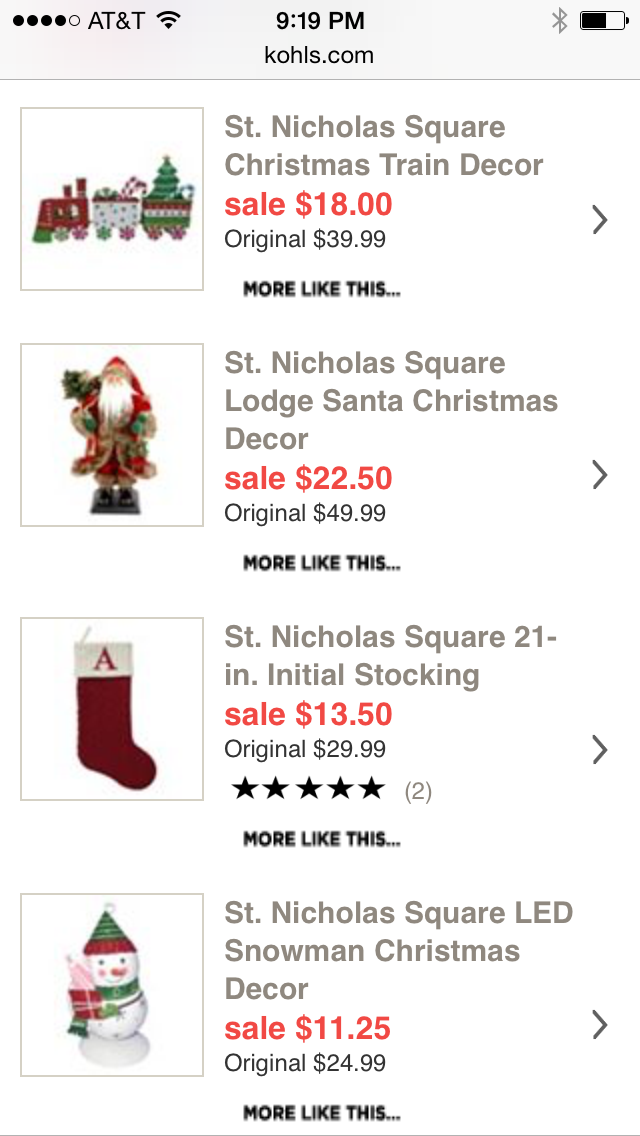The image depicts a cellphone screen displaying the Kohl's website, powered by AT&T. The time is 9:19 PM, with the battery level at approximately 50% and a strong internet connection showing 4 out of 5 bars. The highlighted section of the website features Christmas-themed items from the St. Nicholas Square collection. 

At the top, there is an image of a festive train labeled "St. Nicholas Square Christmas Train Decor," on sale for $18, down from $39.89. Just below, "St. Nicholas Square Lodge Santa Christmas Decor" showcases a picture of Santa Claus, offered at a discounted price of $22.50, originally $49.89. Next is the "St. Nicholas Square 21 inch initial stocking," featuring a red stocking with an "A" on the white cuff, reduced to $13.50 from $29.99. 

Lastly, the "St. Nicholas Square LED Snowman Christmas Decor" presents an image of a box containing a snowman with a green hat and a red rim, holding what appears to be an umbrella, reminiscent of Frosty the Snowman. This item is available for $11.25, marked down from $24.99. At the very bottom, bold black text reads "More like this…" indicating additional similar items available for browsing.